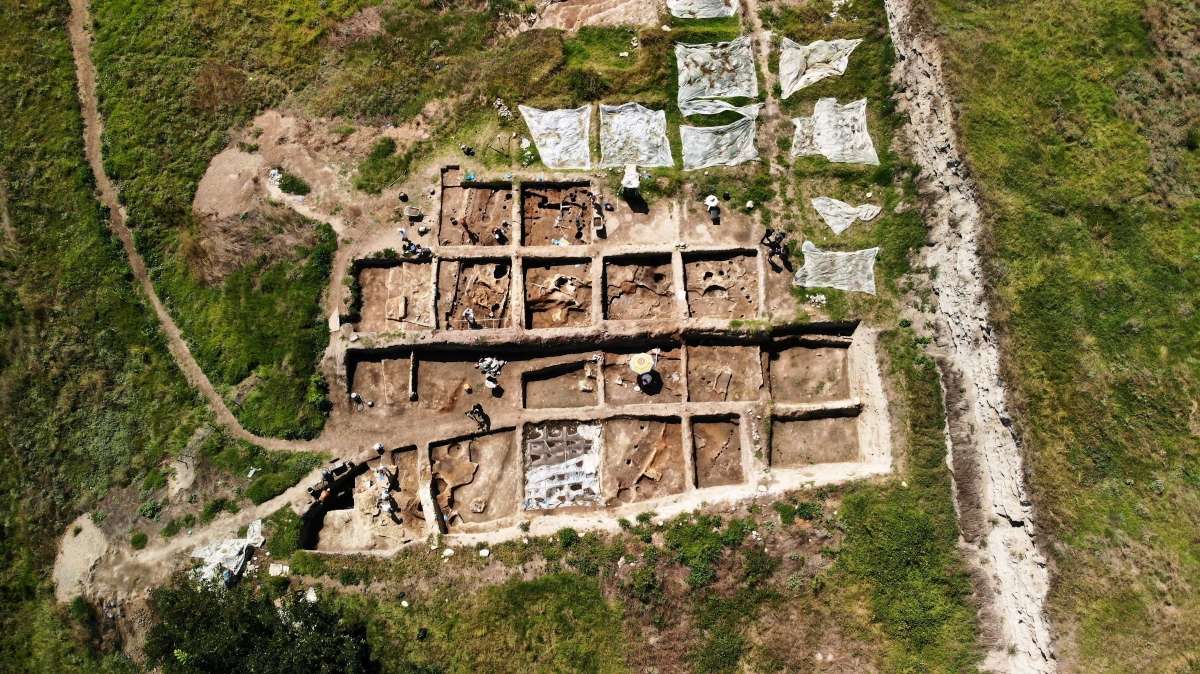The image is an aerial photograph showcasing an archaeological excavation site, prominent in the center with light brown soil and concrete-like structures. This historic site, possibly a fort or a large building, features a grid-like pattern with around 15 to 20 square-shaped plots. The top-down view reveals the intricate layout of the dig, with potential archaeologists visible within some of the plots. The surrounding area is lush and green, indicating a hill or mountain setting enveloped in vegetation. To the left, a path leads to the site, while a dirt road runs vertically on the right side, bordered by a slurry substance. In the upper part of the image, greyish stone-like objects and large white sheets can be observed, adding to the detailed depiction of this fascinating archaeological endeavor.